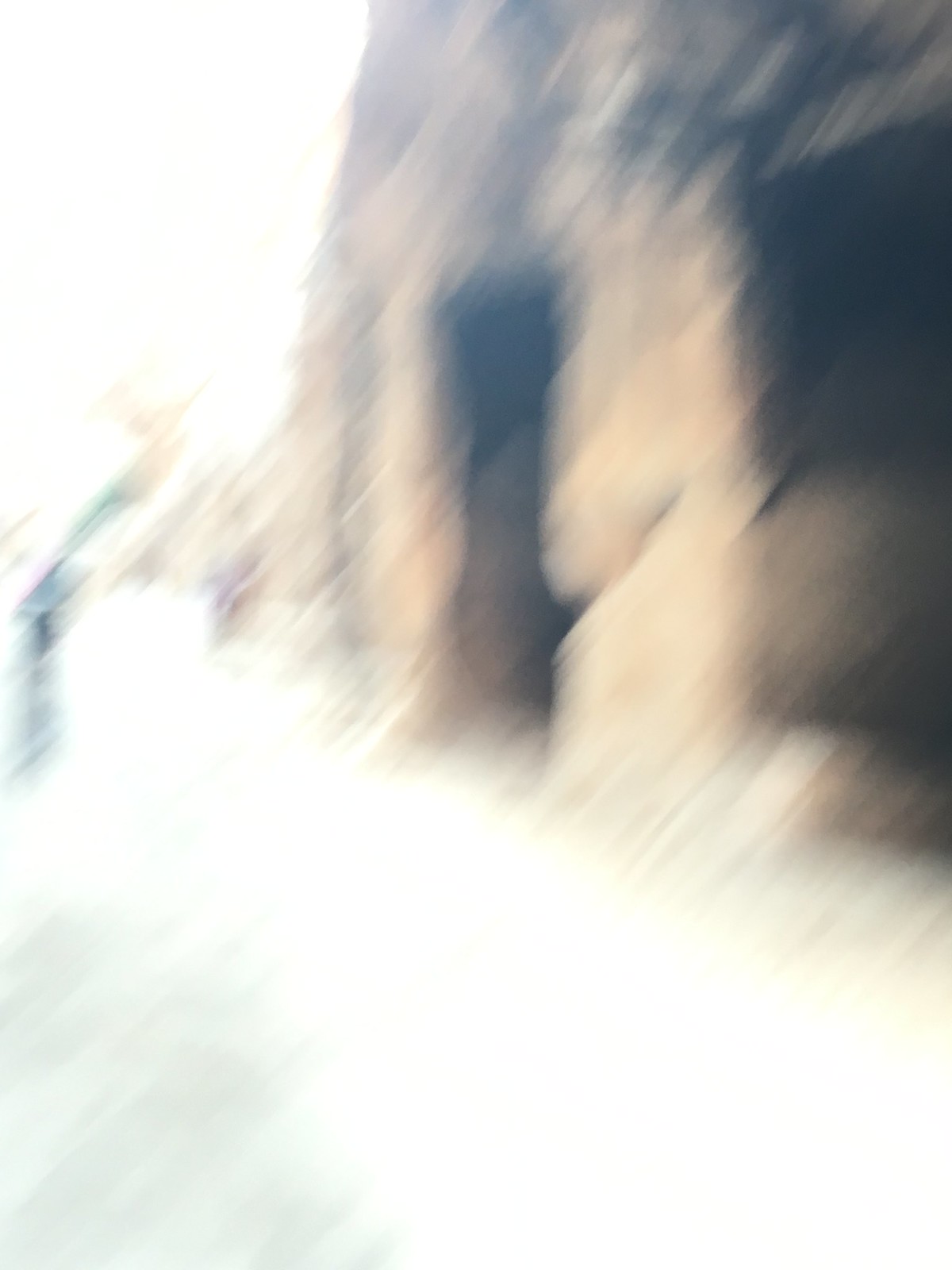A blurred and unfocused image captures a bright, white walkway, intensely illuminated by sunlight, creating significant glare. To the right, a gray stone wall runs parallel to the walkway, suggesting it's part of a building. The structure includes two door-like openings framed in stone, adding to the architectural features. Due to the lack of clarity, it's challenging to discern specific details, but the overall setting appears to be an exterior pathway adjacent to a stone building with multiple entry points.